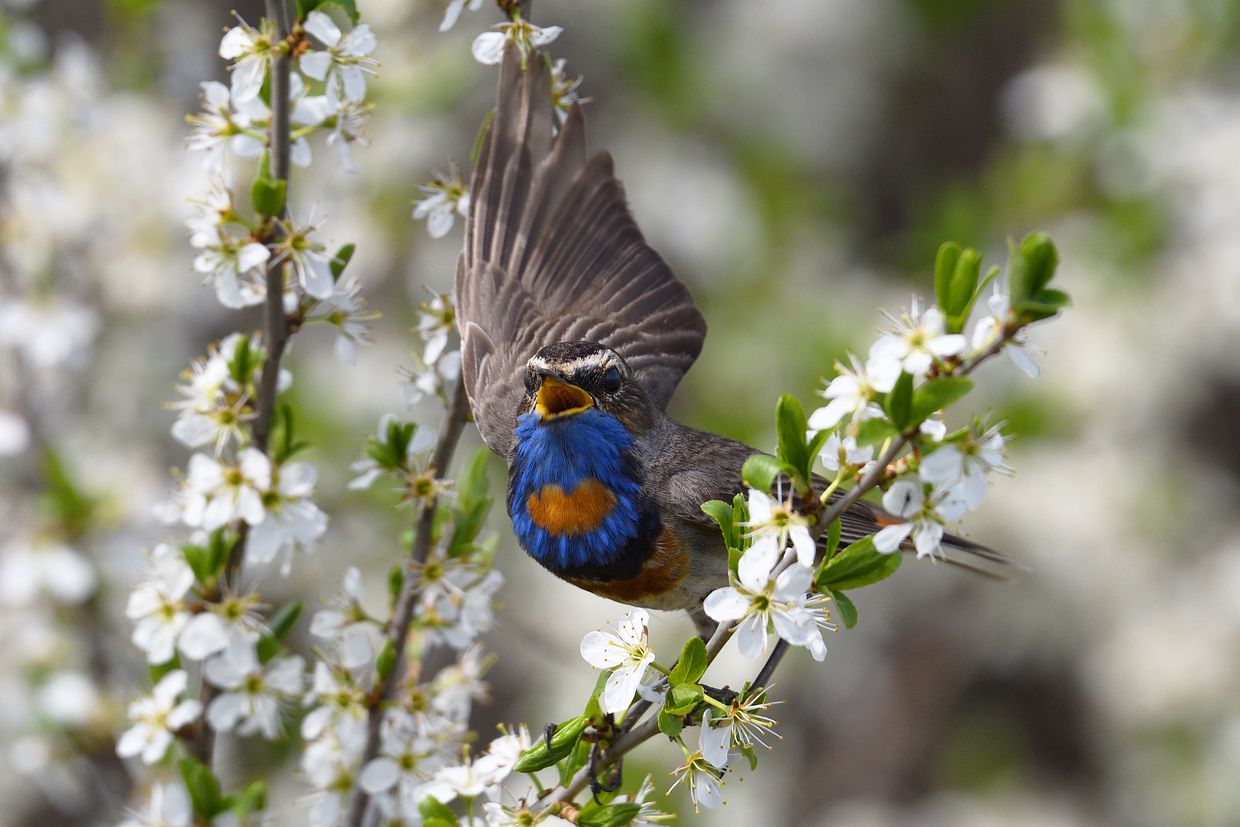The photograph features a striking bird perched on a small, delicate branch adorned with white, five-petaled flowers, which resemble cherry blossoms, surrounded by green leaves. The background is a soft blur of similar flower-laden branches, placing emphasis on the bird in the center. This bird, with its mouth open, has a distinct appearance: its head and part of its belly are a brown-gray color, with a black band around its eyes and a white highlight above them. Its chest features a vivid cobalt blue, accentuated by a heart-shaped marking in a deep orange-yellow hue. One wing is extended as if stretching, while the other remains tucked. The bird has an orange beak and a football-shaped marking of brown on its chest. The top of the bird's body is a light gray, transitioning to brown and white underneath. The image captures the bird perched confidently amidst the white flowers and slender green leaves.